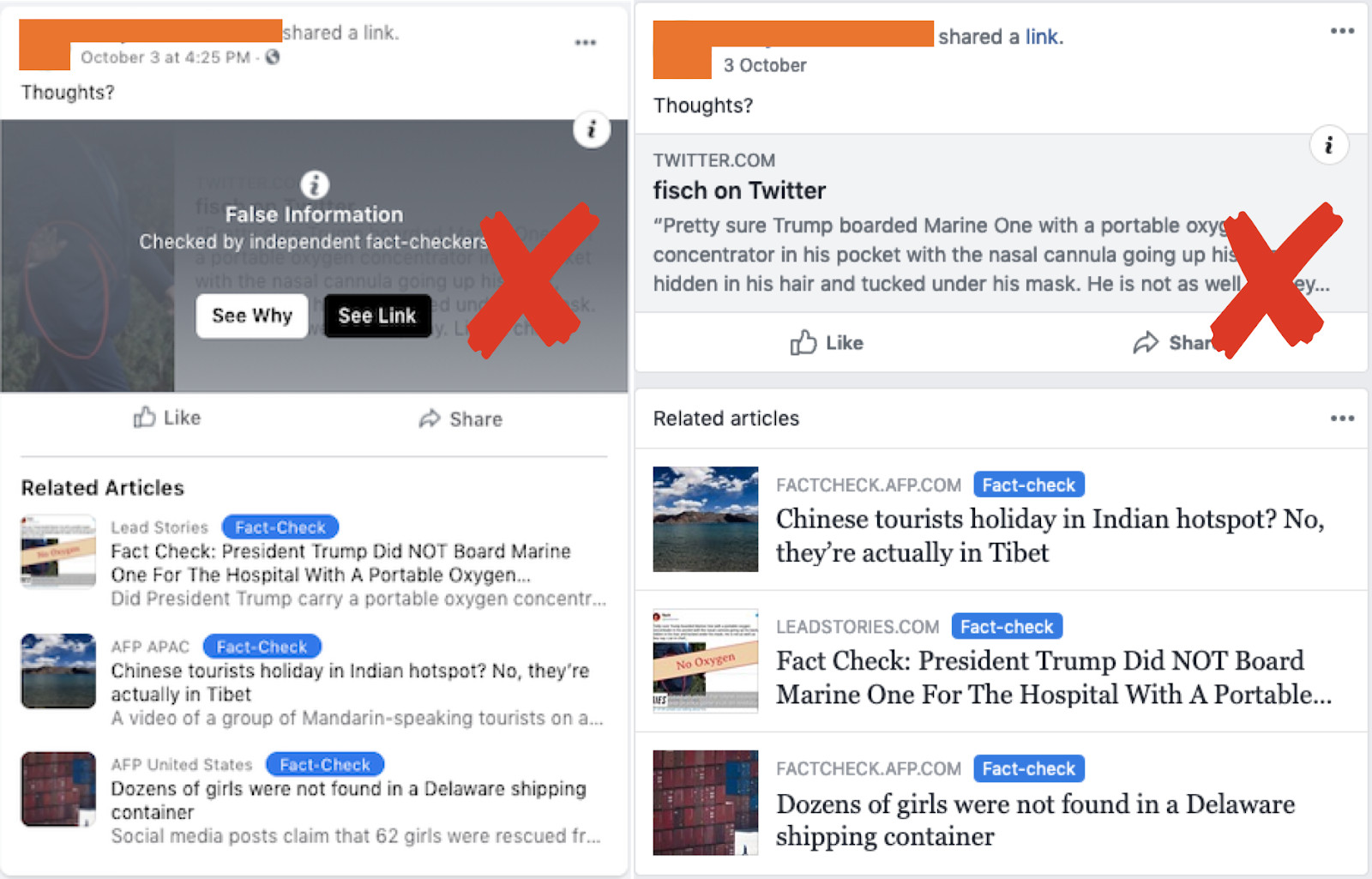This detailed descriptive caption serves to meticulously describe the elements and juxtaposition within the screenshot of the two websites:

"The screenshot features a comparison of two websites displayed side by side. Both websites are marked with a red 'X' indicating some form of error or issue. On the left, the website possesses a dark gray background, whereas the website on the right displays a light gray background. Each screen is adorned with an orange label situated in the top left corner. Beneath these labels, there are three identical pictures showcased on both websites, although they appear in varying sequences. Adjacent to these pictures are blue speech bubble icons, each containing white text, complemented by additional black text on the websites. The upper left of the screenshot is stamped with the term 'False Information,' while the upper right mentions 'Fish on Twitter.'"